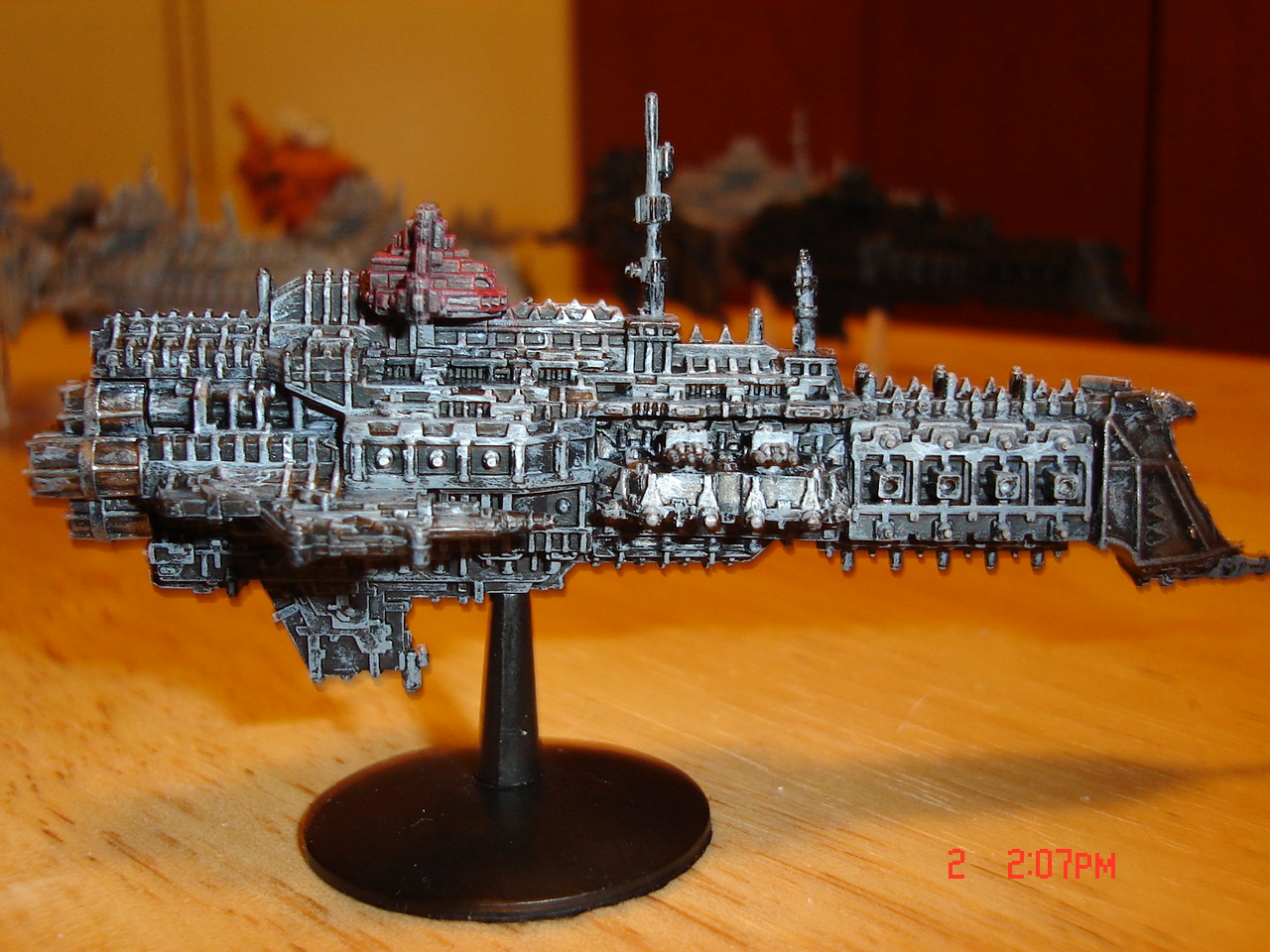The photo features a miniature spaceship model reminiscent of the Battlefleet Gothic series, often used in board games like Warhammer. The futuristic spaceship, predominantly painted in shades of gray and white with subtle red accents, is mounted on a small black circular stand that elevates it, simulating flight or hovering. The stand consists of a circular base with a spike post that supports the ship. The scene is set on a light wooden table, where the wood grain is distinctly visible. In the blurred background, similar spaceship models can be discerned. Notably, the timestamp "2.07 pm" appears in red at the bottom of the image, along with a red object in the background, subtly enhancing the composition's details. The spaceship itself features intricate design elements, including small protruding structures resembling antennas, contributing to its detailed and futuristic appearance.